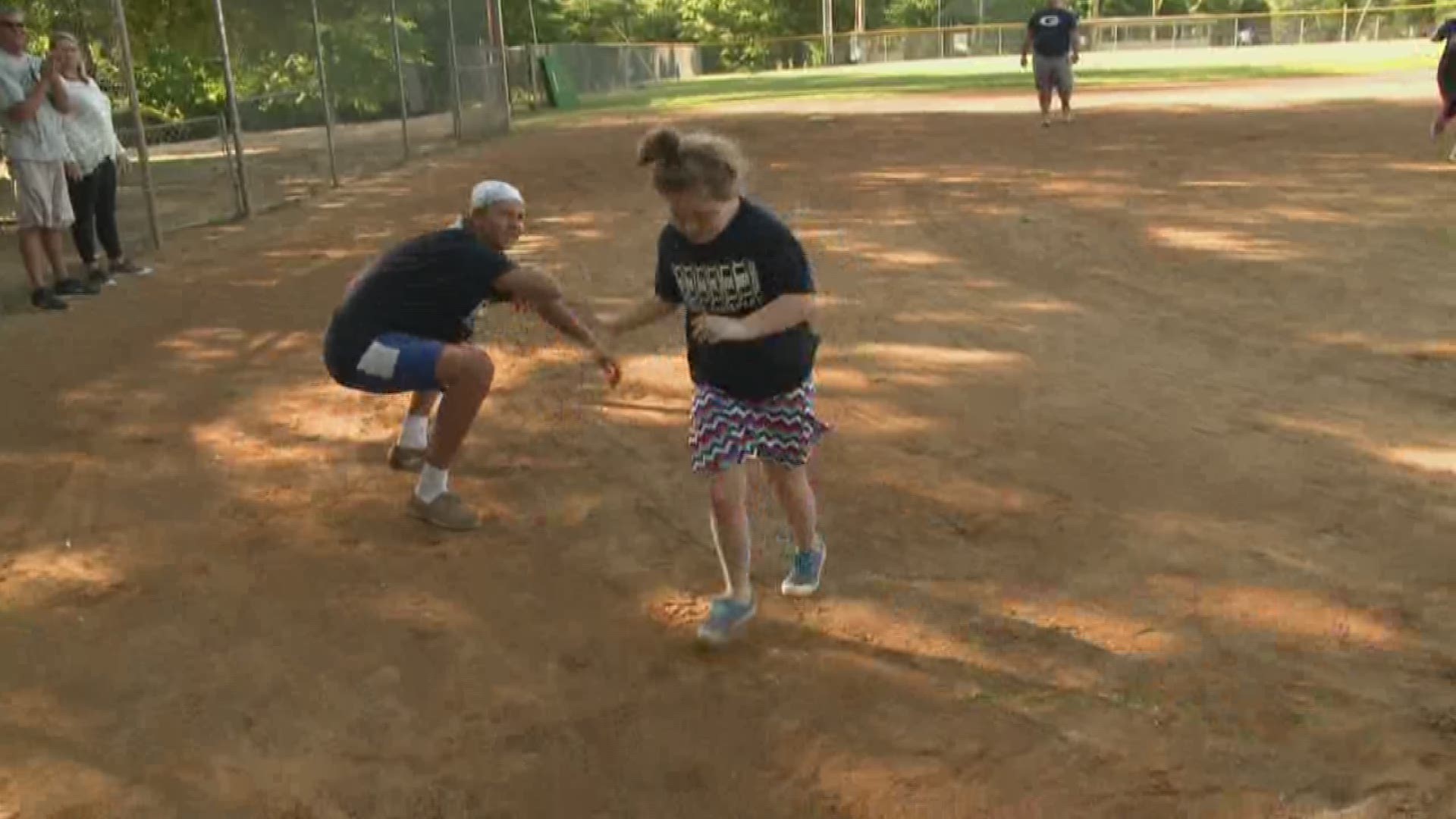In the image, an outdoor park scene unfolds, seemingly capturing a moment of a game or practice session, possibly baseball. Key features include a young girl in mid-action, perhaps running towards home plate, donning a blue t-shirt, a multi-colored skirt with a zigzag pattern in red, white, and blue, and blue sneakers. Her hair is pulled up in a bun. Beside her, an adult male figure, likely in his 30s or 40s, squats down, facing the right side of the picture. He sports a bandana, a black t-shirt, blue shorts with a white pocket, white socks, and brown shoes. 

In the background, a chain-link fence encloses the park area. Leaning against the fence are two observers in the upper left-hand corner. Additionally, another person’s head is partially cut off at the top of the photo. Further in the background, in the upper right-hand corner, another individual is partially visible, with just a bit of their body making it into the frame. The scene transitions from a sunlit background to a shaded foreground, indicating the presence of large, nearby trees. The ground layout shows a mix of dirt in the foreground, leading to grassy terrain beyond the fence, setting a casual yet engaging atmosphere reflective of a community park event.